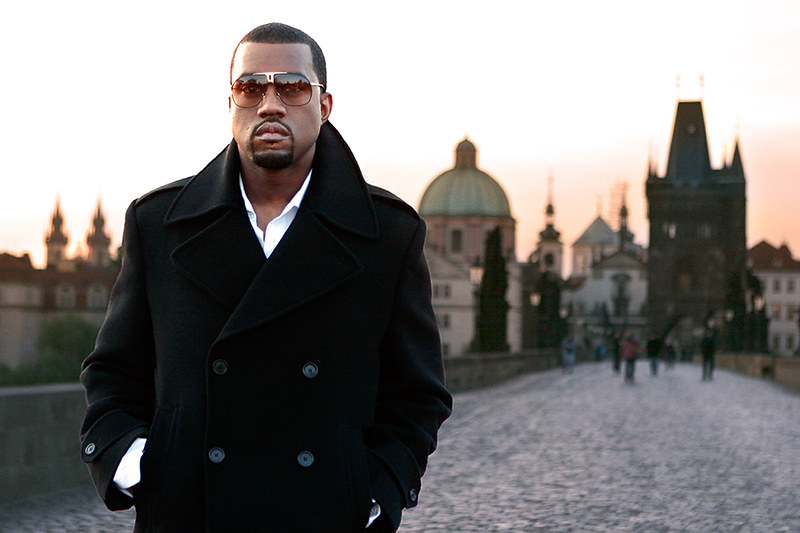In this photograph, an individual who closely resembles Kanye West is the primary focus, occupying the left half of the image. He is captured from the waist up, standing on a pedestrian bridge covered with cobblestones. He is wearing a black trench coat with double black buttons all buttoned up, his hands casually placed in his pockets. Underneath the coat, he sports a white button-up shirt with the top buttons undone. His short hair is neatly groomed, and he has a short goatee. Gold-rimmed aviator sunglasses with brown reflective lenses sit on his face, partially reflecting the setting sun. The bridge is flanked by low brick stone walls, and in the background, a multitude of individuals wander along the bridge, set against a picturesque old European city. The skyline features domed towers and historic buildings, bathed in the warm hues of an orangeish-blue dusk sky, suggesting a time just before nightfall.